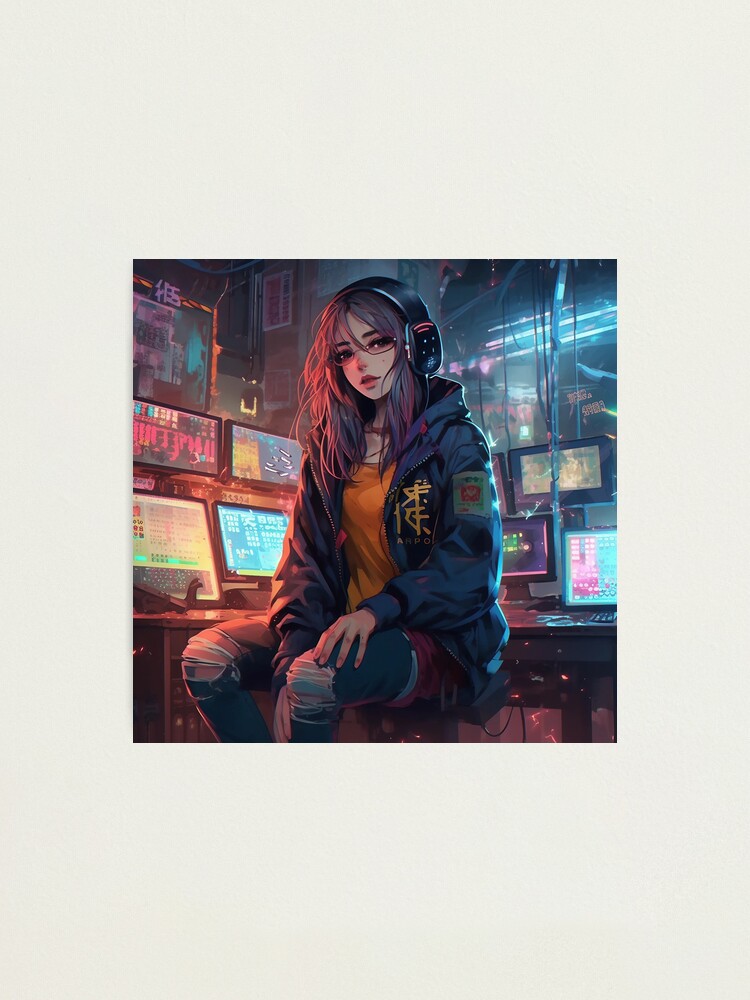This image depicts a young girl sitting on a backless, circular stool in a room filled with various monitors and control panels, reminiscent of a command center. The room is cluttered with six and a half computer monitors of different colors and types, possibly used for monitoring rather than gaming, with some showing landscapes or prints. In front of her is a black desk, above which hangs a large window casting an indistinct view. The room, possibly a basement, is illuminated by fluorescent lights and tangled with numerous wires.

The girl herself is portrayed in a cartoon-like Japanese anime style. She has long, dark hair cascading past her shoulders, and she wears black headphones and glasses. Her attire consists of ripped jeans that expose her knees, a bright yellow top, and a navy blue zip-up jacket with a hood. The jacket features a distinctive Chinese symbol on the left chest area and a green patch with red markings on the upper left arm. Her expression appears indifferent as she remains focused amidst the technological surroundings. The scene is part of a detailed print, mounted with white matting, emphasizing the intricate artistry of the depiction.